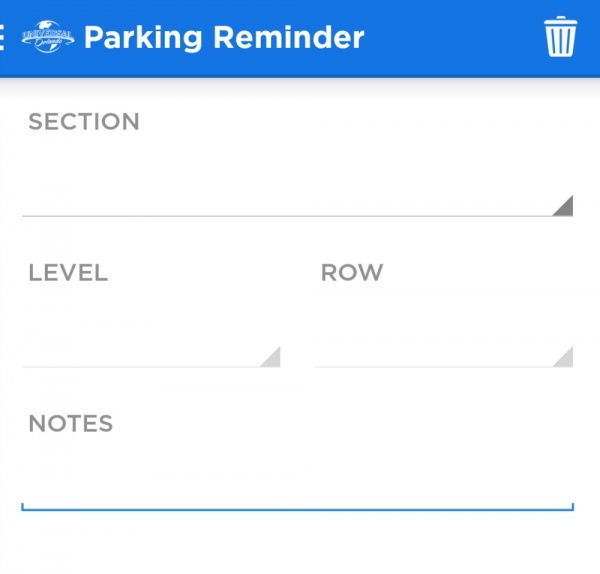The screenshot depicts a parking reminder interface. A blue banner spans the top of the screen, featuring an image of a globe towards the left and the word "Universal." Adjacent to it, prominently displayed, are the words "Parking Reminder." On the far right of the banner sits a white trash can icon.

Below the banner, a gray-titled rectangle labeled "Section" appears. Directly under this is another rectangle divided into two segments labeled "Level" and "Row." Each of these subsections has a small triangle in the bottom right corner, functioning as dropdown indicators; the triangle in the "Section" area is a darker gray, while those in "Level" and "Row" are lighter gray.

Further down, there's a rectangle titled "Notes" for additional information. At the very bottom of the screen runs a wide blue bar, accentuating the interface. The layout is well-organized, with clear sections for different inputs to facilitate easy tracking and reminders for parking details.